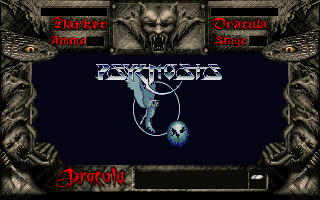Caption:

"This image is a screenshot from a computer screen, likely showcasing the introductory or menu screen of a video game. At the center, there is a prominent black rectangular area. Surrounding this central black space is a border filled with intricate and eerie imagery, including intertwined snakes, demons, and other elements reminiscent of dark, gothic tapestries. At the top center of this border, there is a particularly striking demon’s face with an open mouth and sharp teeth, adding to the ominous tone. On either side of the image, in red font, are the words 'Darker Dracula Ammo Stage.' At the bottom, also in red, the word 'Dracula' is prominently displayed. The middle section features some light blue imagery and text, though it is difficult to decipher exactly what it says. Overall, the image gives off a strong impression of a dark, supernatural-themed video game."